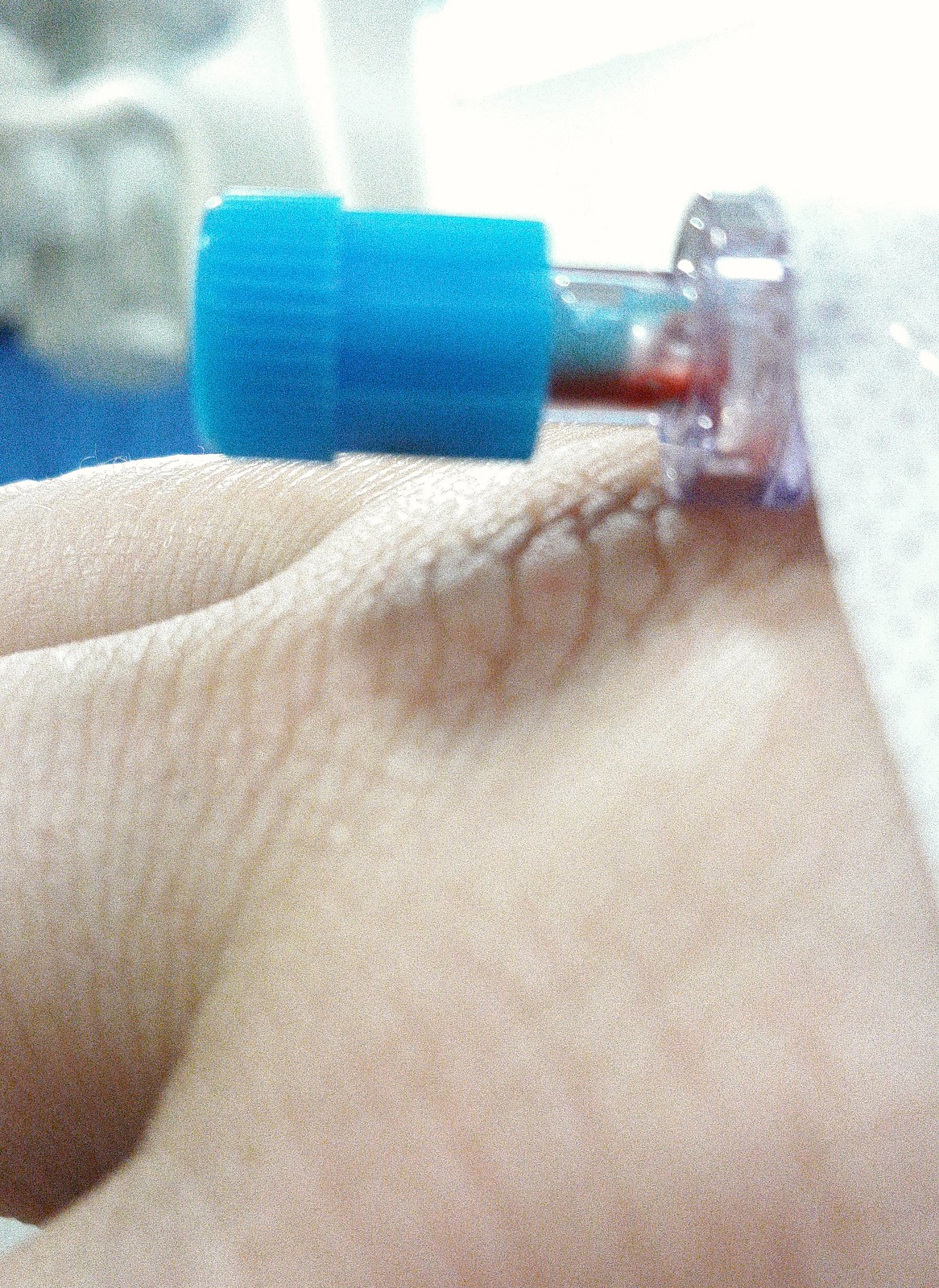This is an extreme close-up view of a hand, specifically focusing on the knuckle area and three visible fingers, likely the forefinger, middle finger, and ring finger. The hand, which has white skin, is fitted with an intravenous (IV) device. The IV setup includes a clear tube with a little blood visible at the bottom, connected to the skin by white medical tape, likely of a cloth type. A blue cap is attached to the device, which could be twisted off to insert a blood collection tube. The background is a harsh, bright light, creating a blurry white and blue haze, possibly indicating hospital lighting and a part of the bed or equipment. The hand is oriented palm-down, emphasizing the detailed wrinkles and lines around the knuckle area.